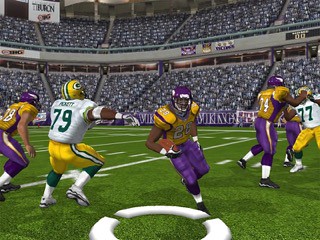The image appears to be a screenshot from a computer game depicting a thrilling moment in an American football match. The stadium is filled with spectators, whose excited faces are visible even in the upper tiers, eagerly watching the action unfold on the field. In the foreground, a player wearing the number 79 jersey stands out clearly.

The players are divided into two distinct teams: one team sports purple trousers paired with yellow tops, while the opposing team is dressed in yellow shorts, green leggings, and white tops. The lush, bright green pitch is meticulously marked with white lines, adding to the realism of the game. A player clutching the ball securely under their arm is seen charging forward, attempting to break through the opposing defense. Several other players are engaged in dynamic tackles, capturing the intensity and fast-paced nature of the sport. The scene is vibrant and immersive, drawing viewers into the electrifying atmosphere of the game.